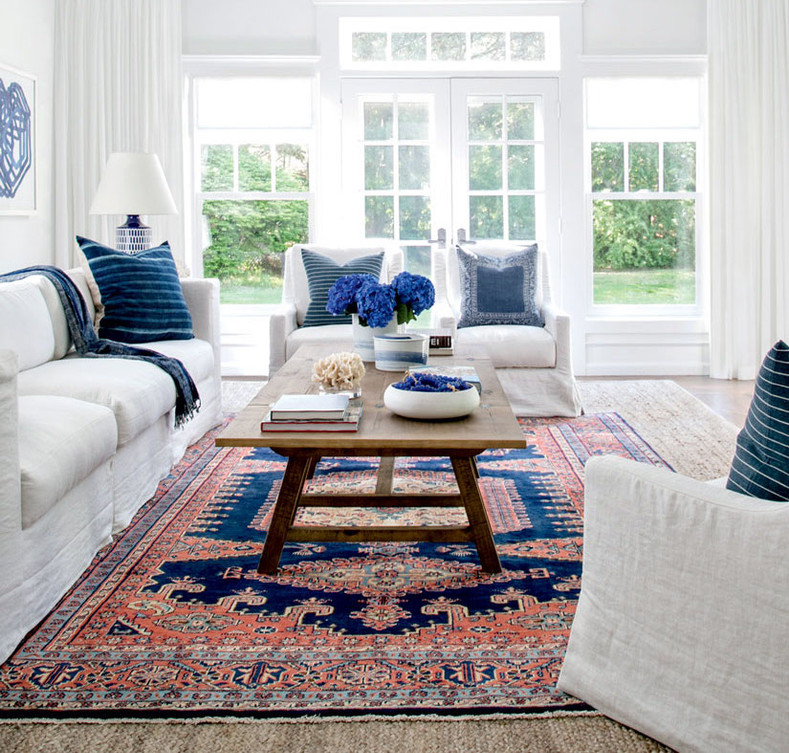The image depicts a bright and inviting living room with a harmonious white color scheme. The room features white walls, white drapes, and white-framed glass windows and French doors, which flood the space with natural light. The furniture includes a three-cushioned white sofa, a white loveseat, and several white chairs, all adorned with navy blue and white striped throw pillows and accented with navy blue throw blankets. A wooden coffee table sits in the center, displaying a white ceramic bowl with blue accents and a vase filled with blue, carnation-like flowers. An oriental rug in shades of peach, navy blue, and various tones of blues and pinks complements the furniture. The coffee table also holds a few books and a piece of coral in pinkish-red. Above the sofa, a piece of artwork featuring blue geometric designs adds a touch of modernity. The room boasts light wood floors and through the large windows and French doors, a lush green yard with trees is visible, enhancing the room’s open and airy atmosphere.